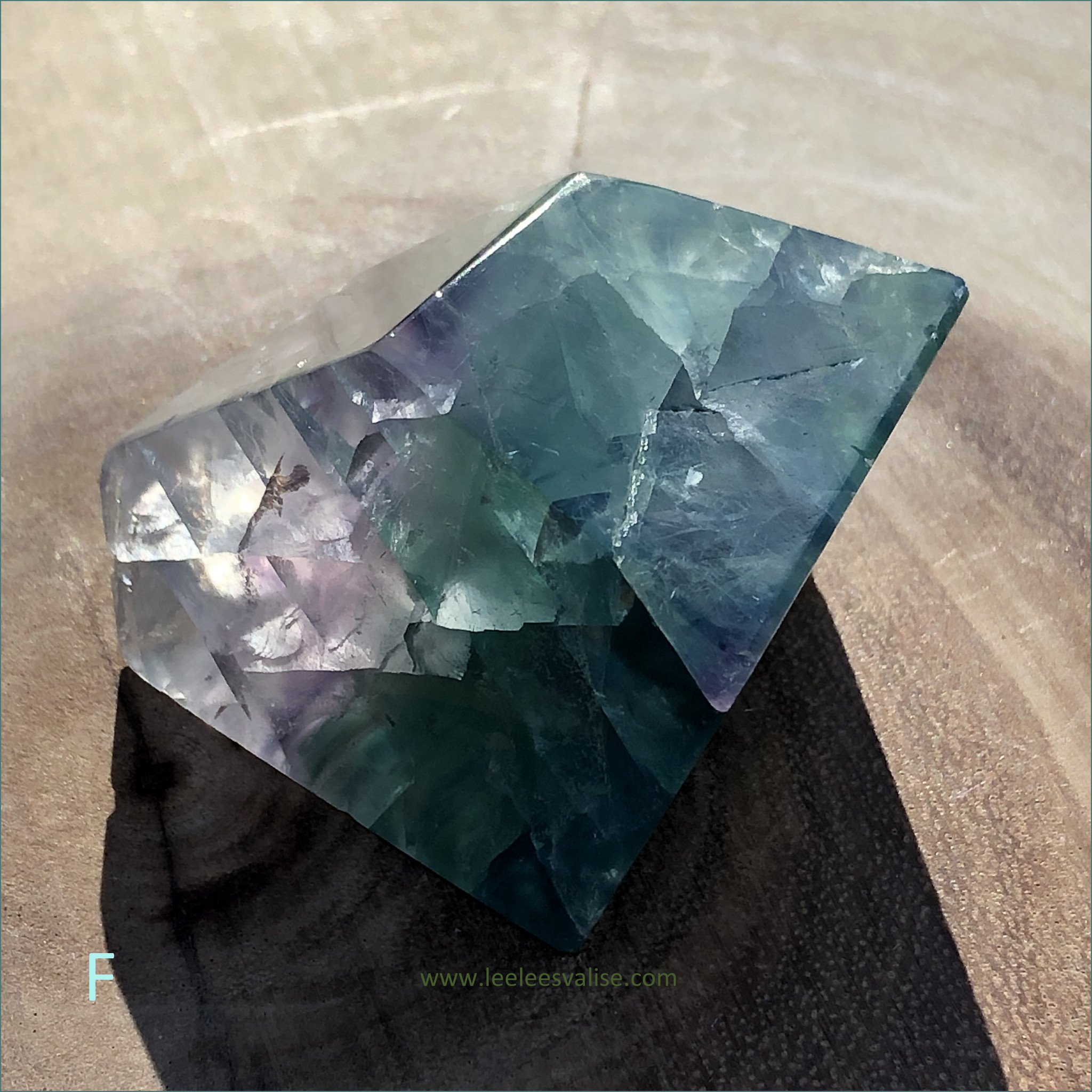The image captures a central focus on a large, smooth crystal, with a grayish-blue hue, standing upright against a completely gray backdrop reminiscent of a cement floor. The crystal, appearing somewhat glassy and rock-like, exhibits smoothly cut surfaces on its diagonal and top sides, showcasing an intricate pattern of different colored crystals within. The object casts a shadow below it, indicating it is illuminated from above by an unseen light source. It rests on a surface that seems to have the detailed pattern of a tree trunk's inside or potentially glass. Notable text in the image includes a blue letter "F" positioned in the bottom left corner, matching the stone's shade, and a web address, "www.liliesvalleys.com," written in yellow at the bottom.